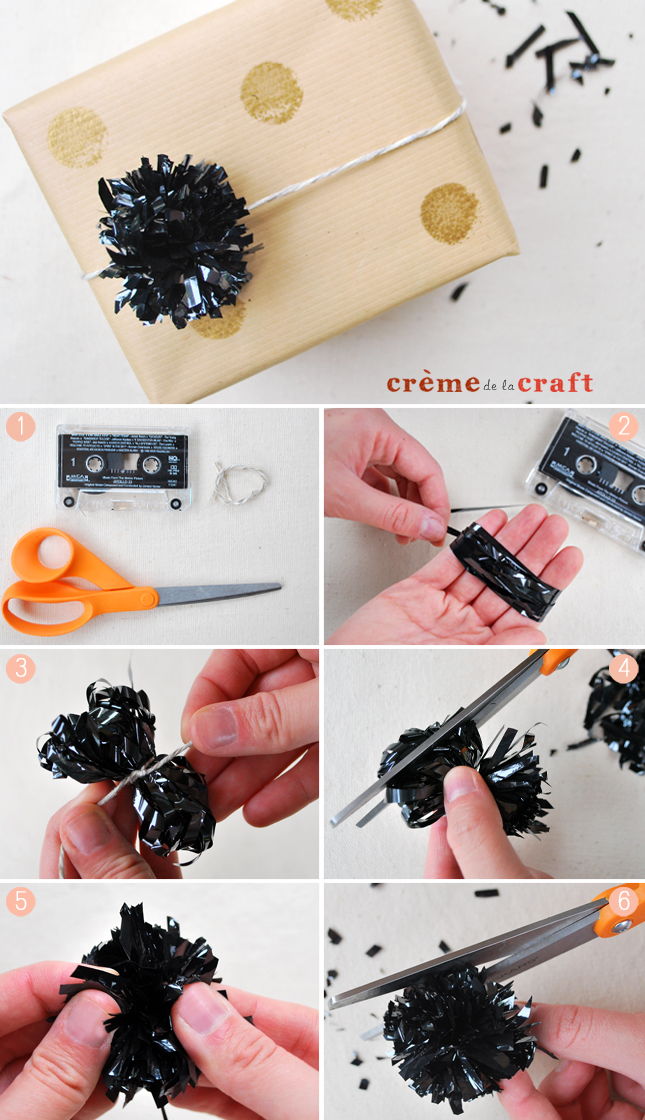The image is a step-by-step tutorial on creating a decorative pom-pom bow from a cassette tape, presented in a seven-photo layout. The largest photograph at the top showcases the finished bow, attached to a tan package adorned with gold polka dots. Below are six smaller images arranged in three rows of two, detailing each step of the crafting process. 

In the first small image at the top left, we see a cassette tape. Below it is a pair of yellow-handled scissors. The right image shows hands pulling out the tape from the cassette. Moving to the second row, the left image depicts the unravelled tape being rolled into a ball with a string. To the right, the scissors cut through the gathered tape. In the final row, the left image features the tape now formed into a poofy ball. The bottom right image shows the ball being opened up and fluffed, completing the pom-pom. 

Step-by-step, this sequence illustrates how to dismantle a cassette, isolate and manipulate the tape, and ultimately fashion it into a shiny, black pom-pom that makes a unique and creative gift decoration.